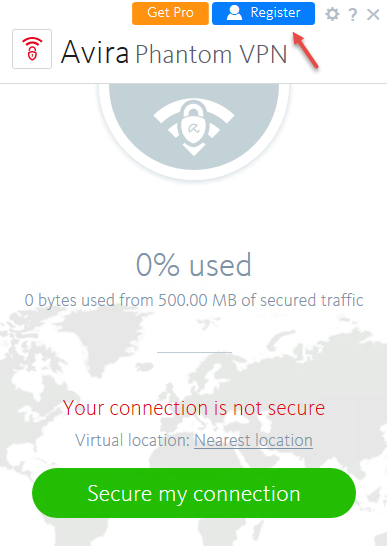The image is a smartphone screenshot displaying a product page for Avira Phantom VPN. At the top of the page, "Avira" is prominently written in black font, with "Phantom VPN" in light gray underneath. To the left of the text is the company logo featuring a red Wi-Fi icon with a padlock at the bottom.

Above the name, there are two buttons: the left button is orange, rectangular, with white text that reads "Get Pro," and the right button is blue, also rectangular, with white text that reads "Register," along with an icon indicating an account.

Beneath this header area, the logo appears again—this time in light gray and white, much larger, and enclosed within a gray circle. The background under this section is white. Further down, in gray text, it states "0% used" and indicates "0 bytes used from 500 MB of secured traffic."

At the bottom of the page, there is a light gray map displaying all the continents on a white ocean background. Below the map, a red warning text states, "Your connection is not secure." This is followed by "Virtual location" in gray text, and "Nearest location." At the very bottom, there is a green button with rounded corners, displaying "Secure my connection" in white font.